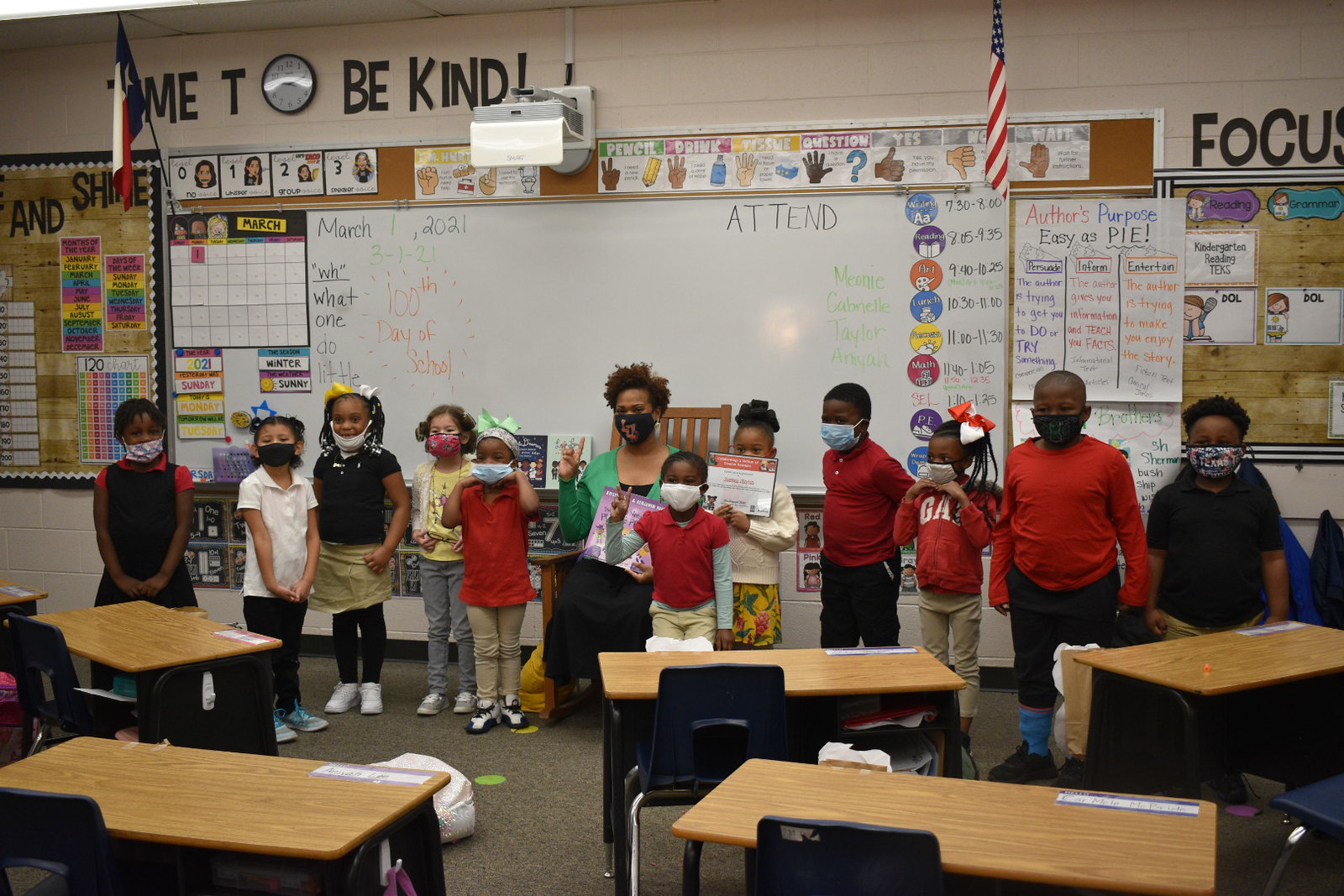Inside an elementary classroom, predominantly composed of kindergarten or first-grade students who are mostly Black, the scene is centered around the teacher. She sits in a wooden rocking chair, dressed in a green cardigan over a black dress, and wears a face mask. The students, also wearing masks, are lined up around her, with one child prominently holding a certificate. 

The backdrop features a whiteboard displaying the date, March 1, 2021, and is flanked by various educational posters and display boards. Above the whiteboard, large letters spell out "TIME TO BE KIND," with the "O" being replaced by a clock. Additionally, a motivational word "FOCUS" is visible on one side. American and Texas flags hang on either side of the display area.

The front of the classroom is arranged with wooden-top desks and small blue chairs, each labeled with the students' names on the upper right side. The students, although masked, appear to be smiling at the camera, contributing to the cheerful and engaging atmosphere of the classroom.